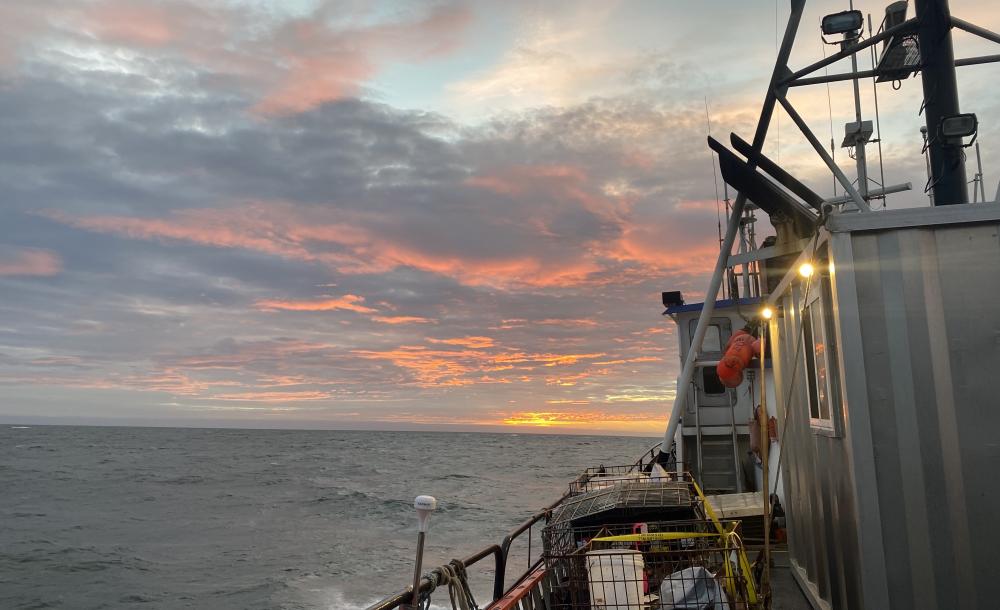A photo captures a serene yet vibrant scene on board a fishing vessel at sea during sunset. The horizon is ablaze with fiery oranges, pinks, and reds, casting a warm glow under the clouds, which are adorned in shades of lavender, orange, pink, and gray. The top of the photo shows a clear blue sky peeking through the clouds. To the left, endless waters stretch out, appearing calm with subtle foam from waves brushing against the ship. The visible part of the vessel, primarily composed of boxy silver structures with corrugated metal, features a cabin with one white window and orange flotation devices attached. Metal crates and buckets are scattered in the foreground, along with assorted fishing gear and rigging. The boat also has some stairs leading to the upper areas, including the captain's booth or steering wheel room. Lights and satellite equipment dot the top of the vessel. A figure in an orange shirt is seen hanging out of a window on the front part of the boat, adding a touch of human presence to the otherwise tranquil maritime setting.